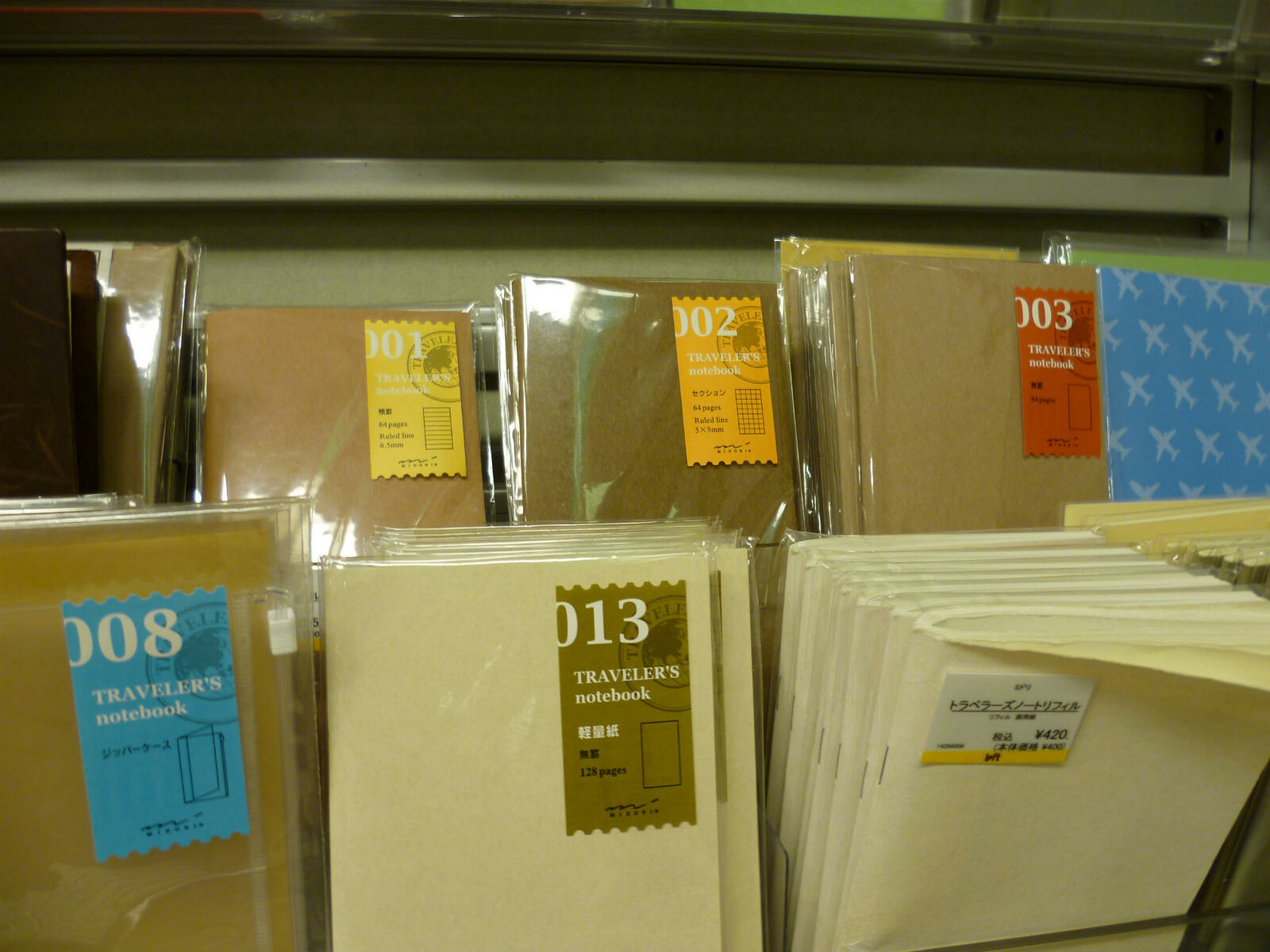This detailed photograph captures a close-up view of a store shelf, most likely in a Japanese stationery store, based on the pricing in yen. The shelf has a metal frame structure with brown boards making up its back wall. Displayed neatly in two rows, the shelf features a collection of Traveler's Notebooks. Each notebook, wrapped in clear plastic packaging, varies in size and boasts covers in various shades of brown, pale yellow, and light brown. On each cover is a branded sticker that reads "Traveler's Notebook" in English, with accompanying Asian text that is too small to decipher, suggesting an additional description or information. The label stickers, varying in color, also display different three-digit numbers, possibly indicating different sizes or model numbers; for example, one notebook shows a blue label with the number 008 and another a brown label with the number 013. Additionally, the front of one notebook is visibly priced at 420 yen. Adjacent to these notebooks is a stack of plain white folders, further suggesting the store's focus on stationery items.